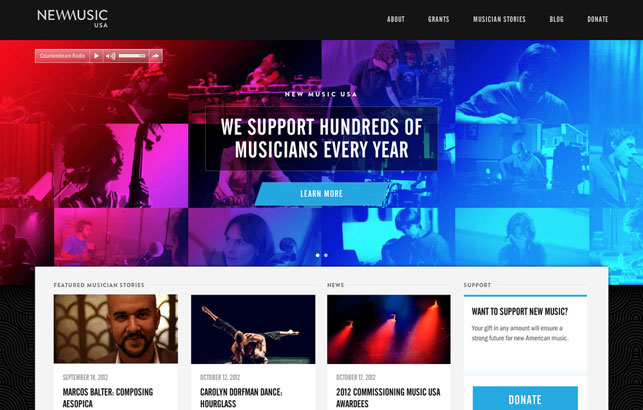The image showcases a website layout. At the very top, a nearly black, dark grey strip spans the width of the page. On the far left in this strip, the words "NEW MUSIC" appear in white, all caps, with "USA" written below it in much smaller, white, all caps text. "USA" is positioned aligning beneath the 'I' and 'C' of "MUSIC." On the far right side of this strip, several navigation tabs are visible, labeled: "About," "Grants," "Musicians," "Stories," "Blog," and "Donate."

Central to the page is a vibrant banner featuring multiple musicians rendered in a gradient that transitions from red to pink, purple, light blue, and dark blue. Within this banner, individual musicians can be seen playing various instruments, including a cello, drums, and a vocalist singing.

Overlaying this colorful banner, a semi-transparent black box contains white text that reads: "NEW MUSIC USA. We support hundreds of musicians every year." Below this text, a blue button with white text invites users to "Learn More."

At the bottom of the page, a section highlights "Featured Musicians Stories" including "Marcos Balter composing Assopica," "Carolyn Dorfman Dance," and "Hourglass and 2012 Commissioning Music USA awardees." A prompt at the end asks, "Want to support new music?" followed by an invitation to donate.